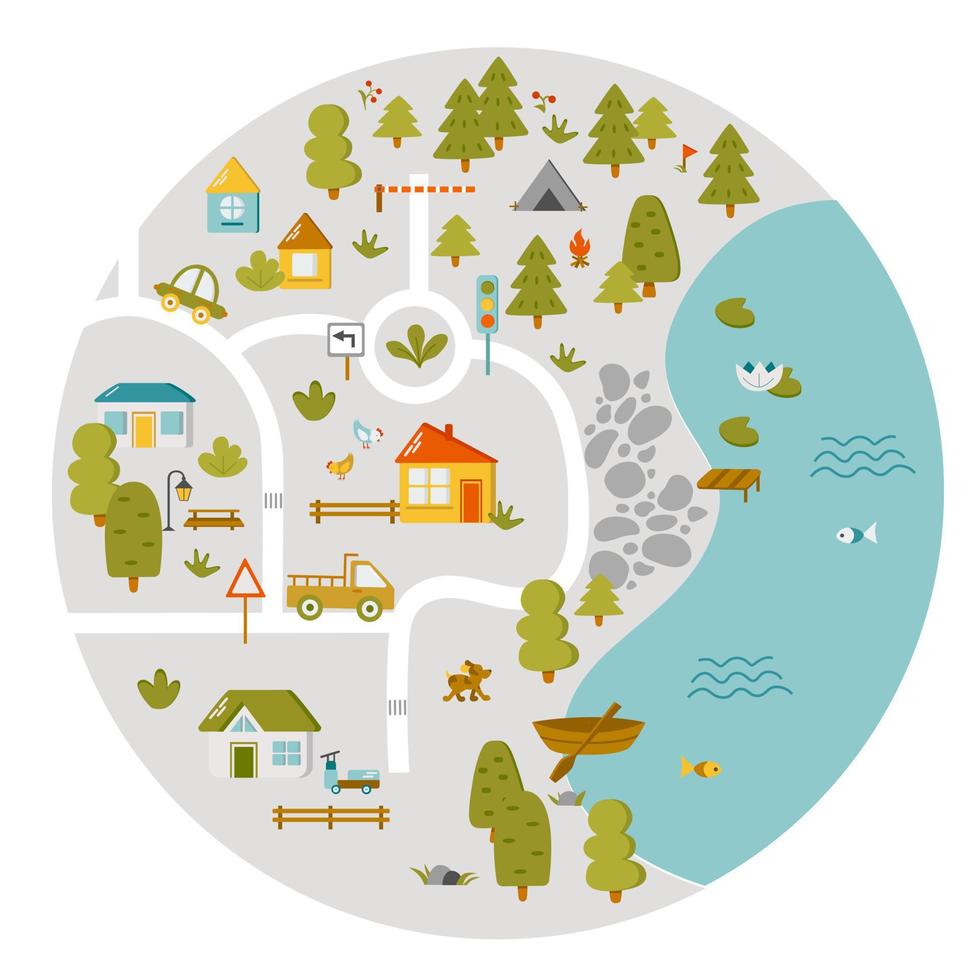This image is a whimsical, bird's eye view map, circular in shape, blending cartoon elements and clip art to depict a quaint small town and its surroundings. On the right side, a large, teal-colored lake occupies much of the space, featuring details like brown rowboats on the shore, a yellow fish and a blue fish swimming, lily pads, flowers, and a small dock. To the left of the lake, the scene transitions into a charming town with white roads snaking through it. Prominent buildings include a yellow and orange house centrally located, a gray and blue house to the far left, and a gray and green house with a green roof towards the bottom left. Between these houses, various roads and pathways connect, one of which curves from the bottom center, loops around near the water, heads up, and curves back around towards the center near the top. In addition to these structures, there are other amusing details such as a dog walking, rocks scattered by the river, and a gray tent nestled among the trees at the top of the image.

The image is also punctuated with various cartoon-style trees, some resembling pine trees, while others are more rounded. On the top left, a church and a picnic table sit among more trees and a car near a street light. Another road from a roundabout connects towards the left forming intersections with other streets. A small farm with chickens, a fence, and a truck can also be seen, enhancing the pastoral charm. The simplistic, yet colorful animations give the image a child-like artistic quality, making it a delightful and engaging pictorial map.